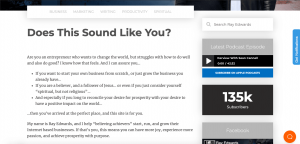The image is a screenshot of a webpage titled, "Does This Sound Like You?" On the right-hand side, the layout consists of six distinct boxes stacked vertically. The top box is a search bar. Below the search bar is a gray box labeled "Latest Podcast Episode." Underneath that is a black box featuring a play button, likely for the podcast playback. Following the black box is a blue box, the content of which is not specified. Below the blue box is a large gray box displaying "135k subscribers." The bottom-most box in the stack is somewhat indecipherable.

At the very top of the screen, there is a long white navigation bar containing five options, though only one word, "Productivity," is discernible due to blurriness. The central portion of the webpage prominently features the title "Does This Sound Like You?" accompanied by a block of text directly beneath it, which is unfortunately too blurry to read. The overall impression is that this is a podcast-related webpage with various interactive elements and sections to navigate through.